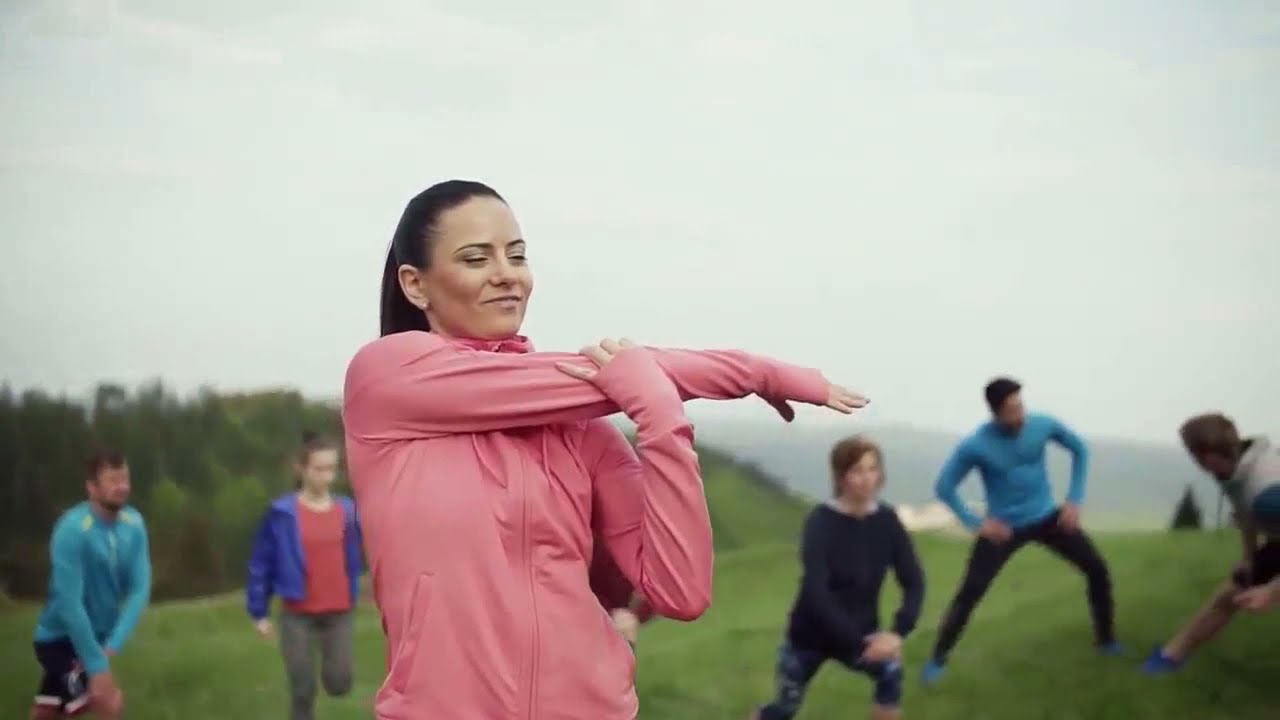In the foreground of the image, a woman in her 30s, with shoulder-length black hair pulled back, is the main focus. She wears a light coral pink zip-up sweater with thumb holes and minimal makeup. She has her eyes closed and a serene, toothless smile on her face. Her right arm is stretched across her chest, and her left hand pulls it towards her body, creating a U shape. Behind her, on a grassy hill possibly overlooking the ocean, five other individuals are visible, though slightly out of focus. To the left, a man in a blue or turquoise shirt and black pants is kneeling or bending, while a girl in a blue jacket and gray pants is raising her left leg. To the right, a woman in a black hoodie squats, focusing on her right leg. Beside her, a man, partially visible, stretches his legs with his hands on his hips, and another man looks on while stretching his own right leg. The background reveals a green field with trees and a cloudy sky, indicating it's not a very sunny day. This scene captures a group getting ready for a jog or exercise session.